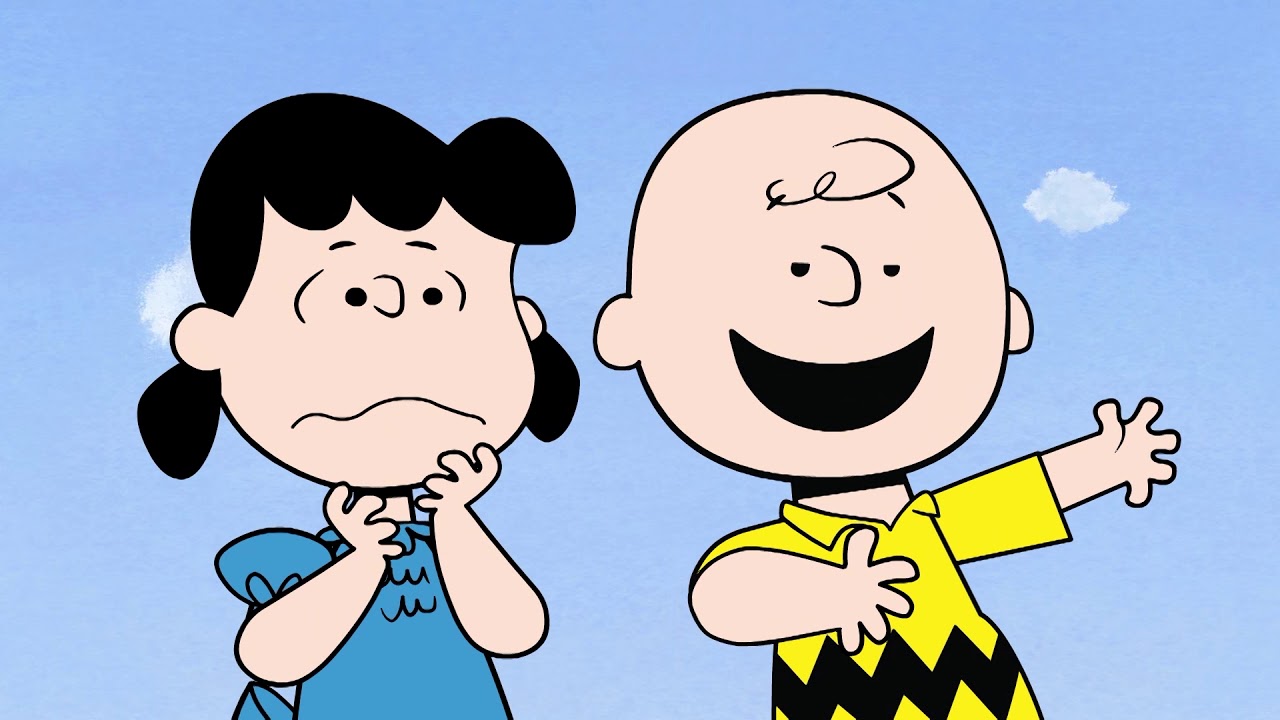The image is a detailed, colorful cartoon illustration in landscape orientation featuring the beloved Peanuts characters, Lucy and Charlie Brown. Set against a light blue sky with fluffy white clouds, the image captures only the upper halves of the characters. Lucy, positioned on the left, is depicted with a confused or dismayed expression, her hands placed under her chin. She has black hair styled into pigtails on either side and wears a blue dress with short puffy sleeves and a blue bow at the back. To her right stands Charlie Brown, characterized by his bald head with a single swirl representing hair. He is smiling cheerfully and points to the right with his left hand, his right hand up near his chest. Charlie Brown is dressed in his iconic yellow shirt featuring a black zigzag pattern across his chest. The illustration conveys a classic scene from the Peanuts series, widely known from both the comic strips and television shows.